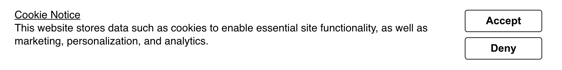The page features a predominantly white background, completely blank except for a small section at the very top. In the top left corner, "Cookie Notice" is clearly labeled in black, underlined text. Directly below this heading, there is a sentence that reads: "This website stores data such as cookies to enable essential site functionality as well as marketing, personalization, and analytics." To the immediate right of this explanatory text, there are two stacked buttons, both with bold, black lettering. The top button is labeled "Accept," while the bottom button reads "Deny." The font used for the "Cookie Notice" heading and the descriptive sentence beneath it is uniform but not bolded, ensuring the main navigation elements are easy to identify and act upon.